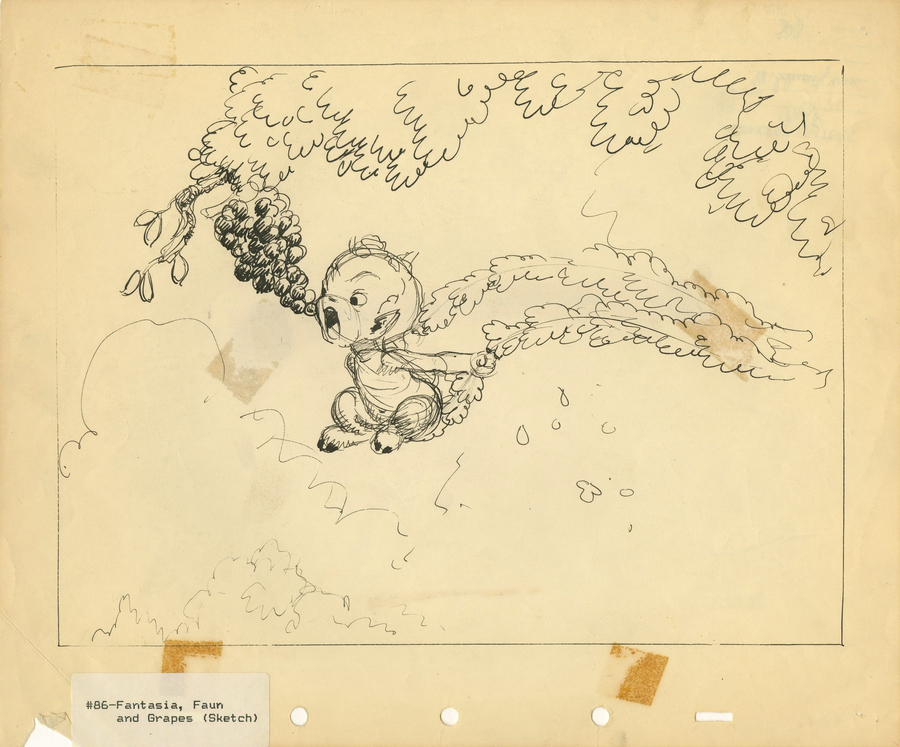The image features an old, worn piece of off-white paper with three binder holes at the bottom and visible tape marks. At the center of the paper is a square pencil sketch titled "Fantasia Fun and Grapes," labeled as #86. The sketch depicts a fantastical creature resembling a baby fawn with hoof-like feet and angular ears, flying through the air on a swing made of branches and grass. The creature has an open mouth, possibly blowing smoke, as it reaches towards a large bundle of grapes hanging from a grassy, leafy tree branch. The detailed smoke or air clouds surround the flying fawn, adding a sense of motion to the hand-drawn scene. Beneath the drawing, a white label with black text reads "86-Fantasia Fawn and Grapes" with quotation marks around "sketch."